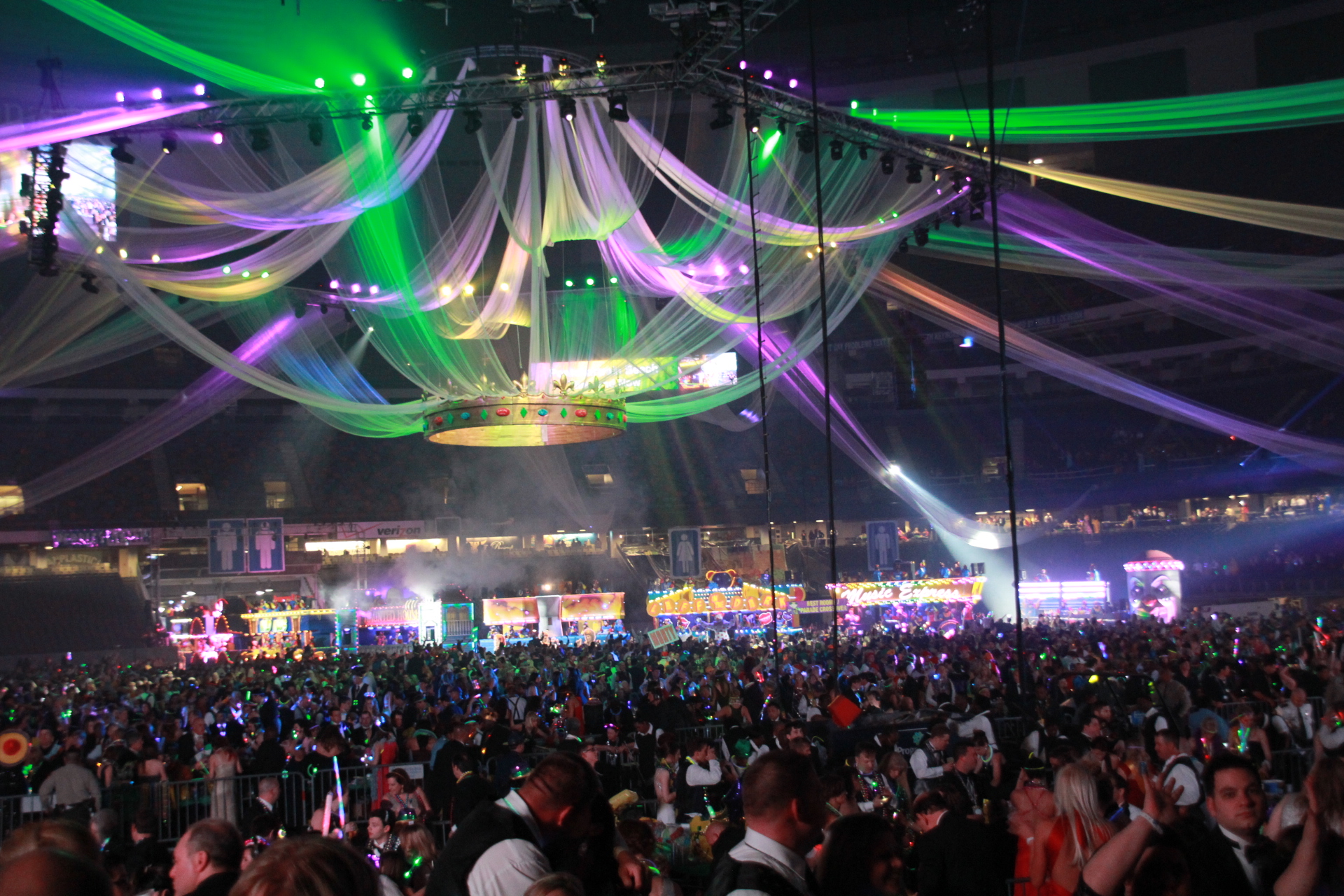This image captures the vibrant and electrifying atmosphere of what appears to be an indoor rave or dance club event. The space is dimly lit, with illumination provided by an array of colorful lights, including lasers and neon strips hanging in a circular formation from the ceiling. This creates a mesmerizing visual effect with hues of green, purple, yellow, orange, cream, white, and pink casting dynamic light patterns across the scene. Below, a dense crowd of possibly thousands of people, some wearing tuxedos and vests, is tightly packed, dancing and moving to the beat. The background features additional structures, possibly booths or shop fronts, outlined in neon lights. On the left side, a large screen and a sign resembling a restroom indicator add to the complexity of the scene. Overall, the spectacle of lights and the massive crowd suggest a highly popular event, pulsating with energy.